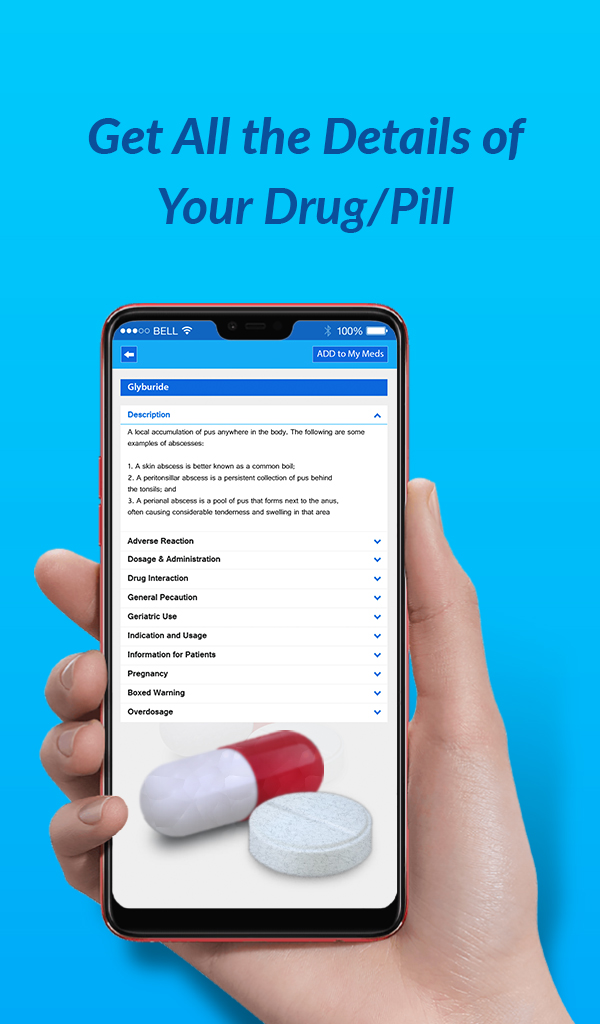The image showcases a rectangular cell phone against a light blue background. Emerging from the bottom right corner, a hand with visible thumb and four fingers holds the phone, displaying its screen prominently. The palm is facing forward.

On the screen, the status bar at the top indicates "Bell 100% battery," highlighted in blue. Below this, a blue title strip reads "GLYBURIDE." The displayed text pertains to a drug, describing a local accumulation of pus anywhere in the body, followed by examples and details about abscesses.

Further information is organized into columns labeled: "Adverse Reaction," "Doses and Administration," "Drug Interaction," "General Precaution," "Geriatric Use," "Indication and Usage," "Information for Patients," "Pregnancy," "Box Warning," and "Overdoses." Adjacent to this text, there is an illustration showing the drug in two forms. One form is a white and red capsule, and the other is a grayish, scored, round pill.

The background of the phone's screen is white, enhancing the clarity of the displayed information.